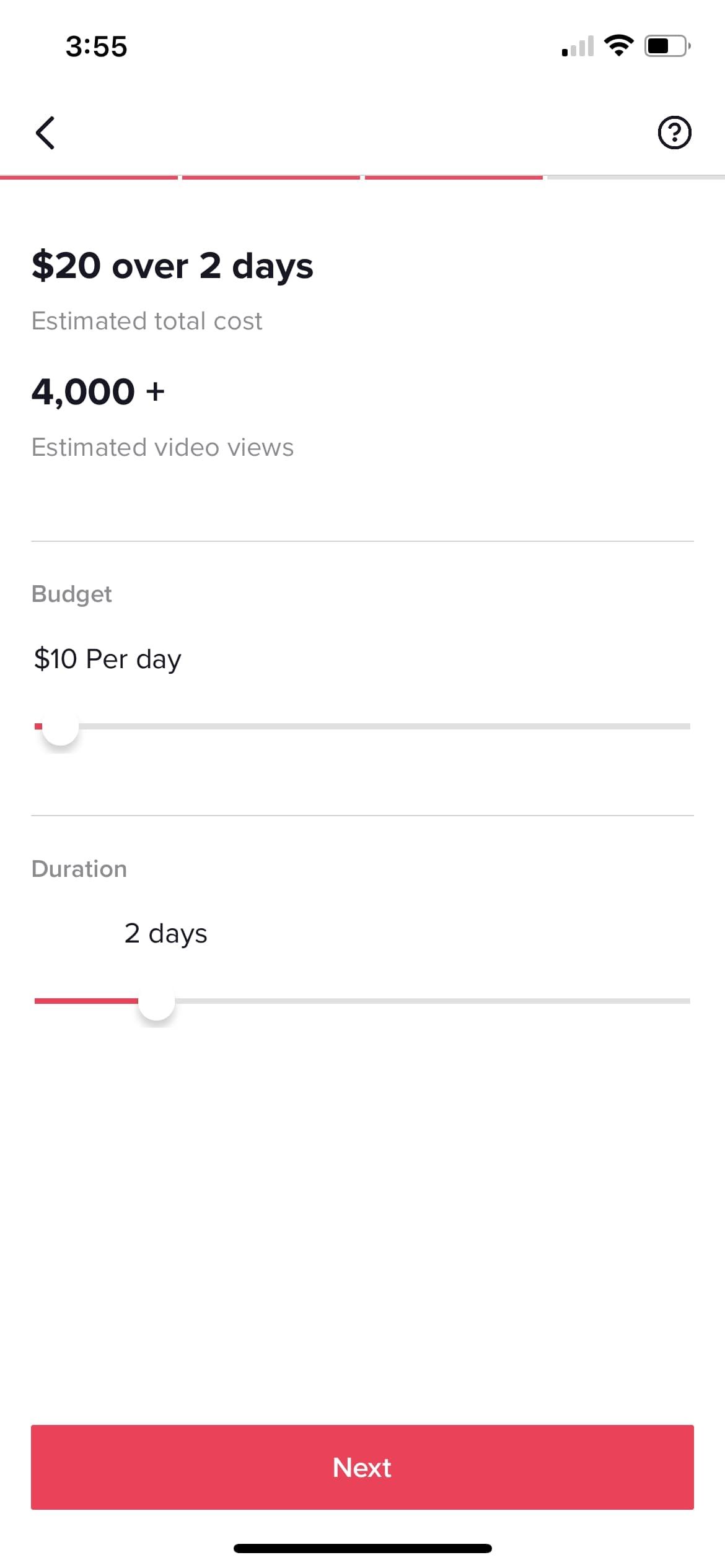This image depicts a mobile phone screen showing an app interface, possibly for setting up an advertisement. The status bar at the top displays full connectivity, battery life, and the current time of 3:55. The screen is divided into two main sections. 

The upper section shows a progress indicator with its title "Estimated Total Cost," suggesting the user is setting a budget for an ad campaign. Below this are four small progress bars, where three are filled in red, indicating completion. The caption reads $20 over two days, and an estimated total cost exceeding 4,000 video views. 

The lower section is split into two components: "Budget" and "Duration." The "Budget" section has a slider set slightly to the right, increasing the daily budget to $10, as indicated by the slider's red fill. Similarly, the "Duration" section slider is set to two days, with the red portion showing the selected timeframe. 

Below the sliders, a prominent red rectangular button labeled "Next" in white text is visible, inviting the user to proceed to the next step. At the very bottom of the screen, a narrow black bar completes the phone's display, marking the end of the ad setup interface.